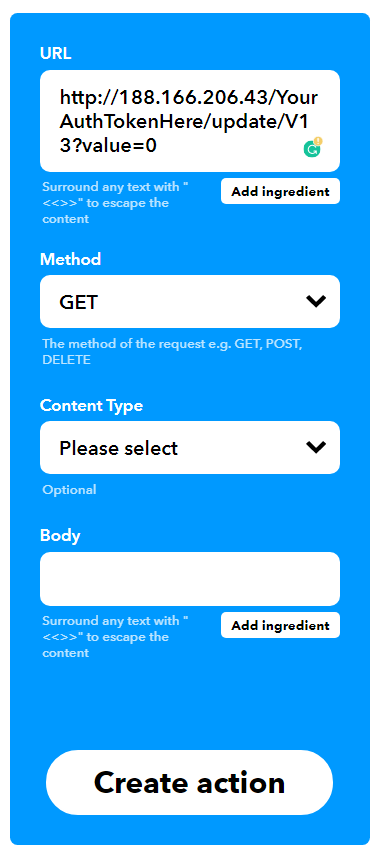This image depicts a user interface for setting up a web request. The interface is housed within a bright blue rectangular area. 

At the top, white text labeled "URL" is prominently displayed. Directly below this label is a white text box containing an HTTP address in black text. To the right of this text box, there is a smaller white button labeled "Add Ingredient" in black text. 

Underneath the URL section, a white instructional text suggests "Use back and forward arrows to navigate content."

Following this, there is a "Method" section labeled in white text. Here, a white drop-down box includes a "GET" option and features a black downward arrow on its right side. Below this, a white instructional text defines "GET, POST, DELETE" as potential request methods.

The next category is labeled "Content Type" in white text. Below it, a white rectangular drop-down box displays "Please Select" in black text, accompanied by a downward arrow icon.

The final category is labeled "Body" in white text, featuring a blank white rectangular text box for user input. To the right of this text box, there is another small white button labeled "Add Ingredient" in black text.

At the bottom, a central white oval-shaped button with black text reads "Create Action."